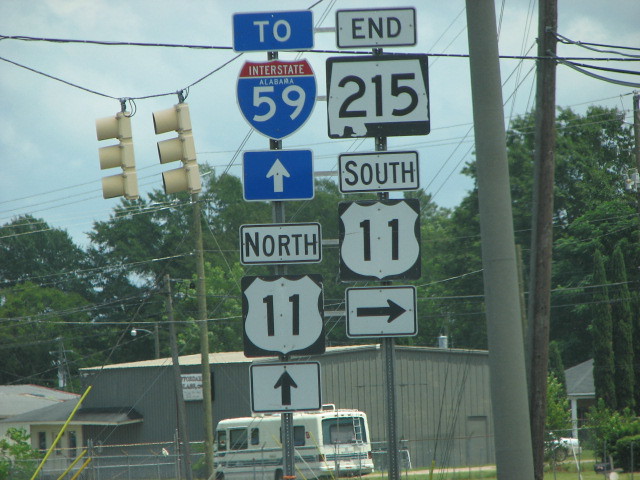The image depicts a bustling street scene in an American city during the daytime. The sky is a light blue, dotted with white clouds, creating a serene backdrop for the organized chaos below. Road signs are stacked atop one another in two columns, an eye-catching jumble of directional instructions. The left column of signs reads from top to bottom: a blue metal sign with the number "2," followed by a shield-shaped sign featuring "Interstate 59" with "Alabama" inscribed between "Interstate" and "59," and an upwards arrow indicating "North 11." The right-hand column features an upwards arrow with the word "End," below which there is "215," "South," "11," and a rightward pointing arrow.

Traffic lights add to the scene’s complexity, hanging amid the sea of signs. In the background, a row of trees stands tall, framing a grey building whose construction materials suggest wood or tin or another type of metal, perhaps giving it an industrial feel. A white minibus or campervan, adorned with green lines and a green window surround at the back, adds a touch of color and indicates travel or tourism.

The overall scene is one of dynamic urban life, where the convergence of signage, transportation, and infrastructure creates a vivid tableau of everyday America.